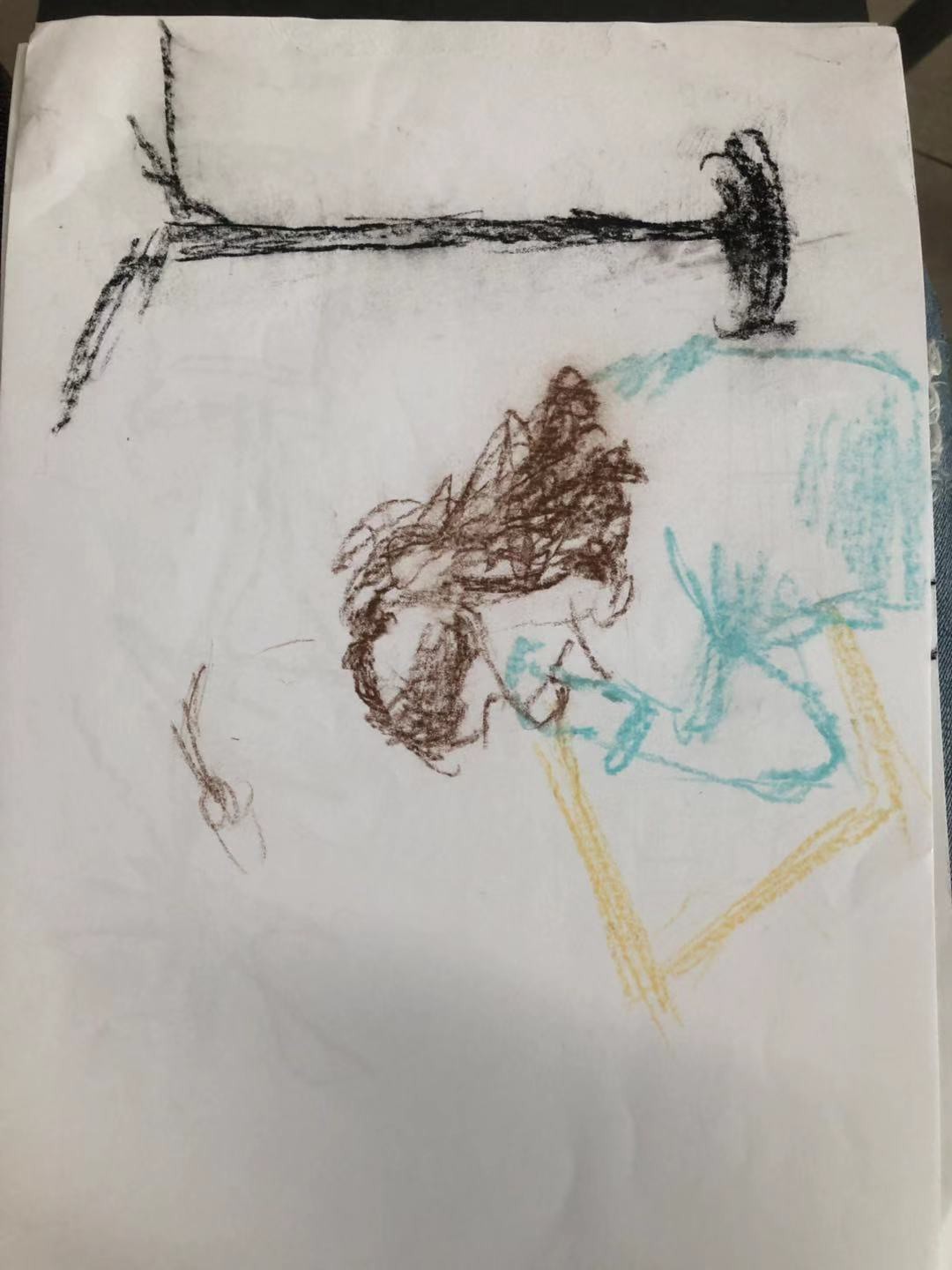The image depicts a child’s crayon drawing on a plain, vertical white piece of paper. The drawing features a black horizontal line at the top with branching black lines, which gives the appearance of a lamp or a light post with two arms. Below this, there's a light blue crayon scribble that suggests a person's blue clothing. Underneath this blue area is a half-square, colored yellow, that resembles a desk or a surface. On the left side of the page, the drawing includes a figure with brown curly hair flowing down to the shoulders, suggesting a person possibly sitting at the desk, with arms bent at the elbows, indicated by the blue crayon marks. There are additional brown scribbles to the left of the figure, adding more detail to the scene. Overall, the drawing seems to represent a person with a blue shirt and brown hair, possibly interacting with objects on a desk-like surface, all under the semblance of a tall, black, branching structure.